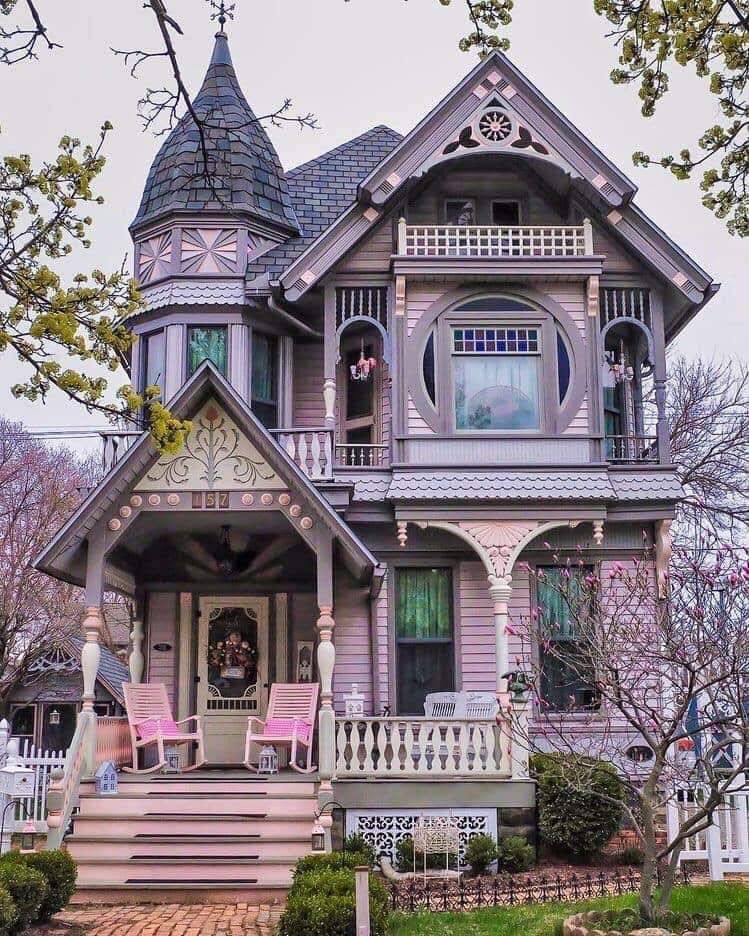The image depicts a charming and whimsical gingerbread-style house with a lavender and pink façade. The three-story structure features a variety of intricate decorative wood trims and cutouts, giving it an old, fairy-tale-like appearance. A turret on the left side presents an octagonal shape with a pointed spire roof. The main entrance is accented by a large peak roof adorned with paintings of flowers and trailing vines. 

The house’s roof sports gray shingles in varying shades. Steps lead up to the covered porch, which houses two pink rocking chairs with matching pillows and a white bench. The fenced-in area of the porch provides additional seating. Below, there is a brick foundation seen at the base. 

In the yard, a neatly arranged circle of bricks encloses a small grassy area with several foot-tall shrubs and a small tree bearing pink flowers. The scene also includes another pink-flowered tree in the distance. The bright but gray, clouded sky serves as the backdrop, with green-leafed tree branches framing the upper corners of the image, enhancing the overall enchanting ambiance.